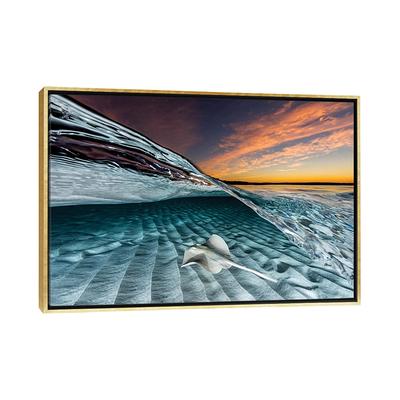The image displays an elegant framed canvas painting, likely a print, commonly seen on e-commerce websites like Amazon, Wayfair, or eBay. The thin frame appears to be made of a gold or natural wood finish. It is slightly tilted, with the left side sticking forward more than the right. The artwork itself depicts a beautiful and serene ocean scene during sunset. On the right side, the sky transitions from a golden hue at the horizon to blue, blending into white clouds above. As the sun sets, the scene darkens with rich blues and browns, evoking the onset of night. The bottom half of the painting features clear, turquoise ocean water with waves gently rolling over rippling white sand. A light gray stingray can be seen swimming gracefully in the water, adding a touch of life to the tranquil landscape.